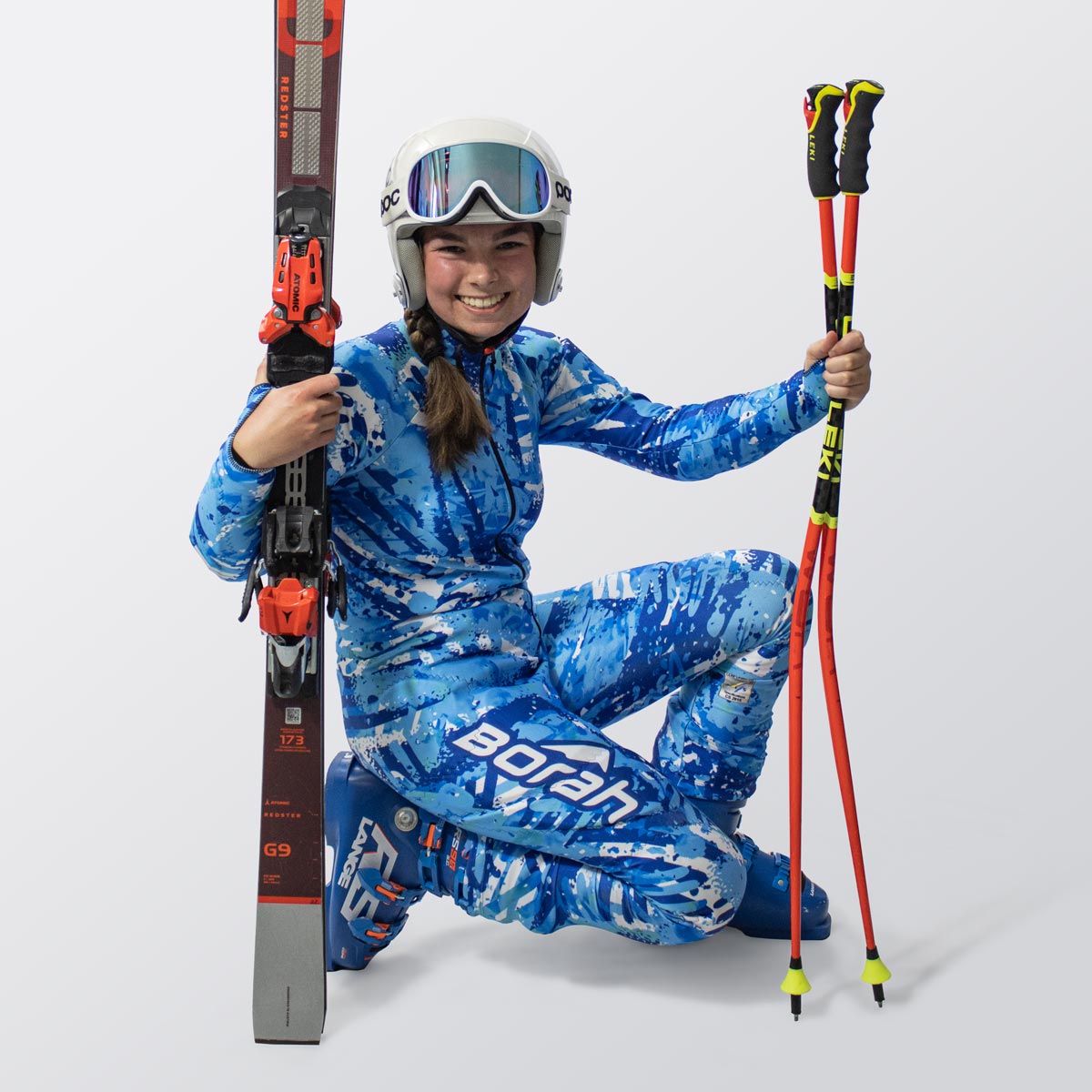The photograph is a square image featuring a young Caucasian woman, with her face visible and smiling, set against a seamless white background that provides no distinction between the floor and the wall. The woman is kneeling on her right knee, with a shadow underneath indicating it doesn’t fully touch the ground. She is dressed in a single-piece blue, white, and dark blue camouflaged jumpsuit, with a black zipper running down the front and a tall collar zipped up. The jumpsuit has thumb loops at the end of the sleeves and white lettering on the right thigh that reads "Bora". She is wearing large blue plastic boots secured with blue and orange clasps, which have "RS Lange" written in white letters on the side.

Her brown hair is styled into pigtails that peak out from under a helmet, which is equipped with blue reflective goggles perched on top. In her left hand, she holds red ski poles with black handles, and in her right hand, she holds skis that are predominantly black and red with some gray on the lower part. The woman exudes a professional demeanor, indicated by her confident pose and equipment, suggesting she is an experienced skier.